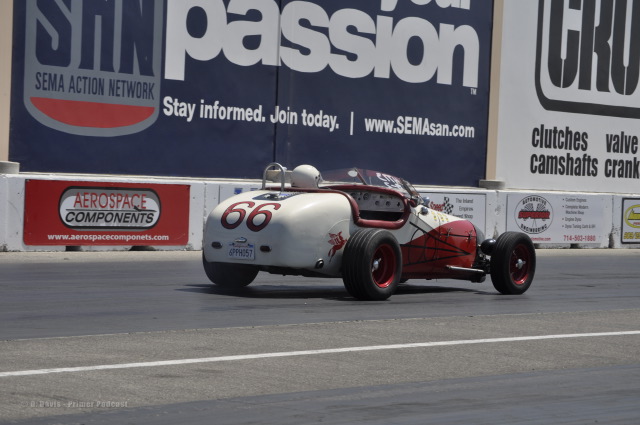The image captures a daytime scene at a modern racetrack, showcasing a nostalgic motor racing event. The racetrack is primarily asphalt with white markings, flanked by barricades adorned with numerous advertisements. The central focus is a distinctive white and red race car, sporting a retro design reminiscent of the 1950s or 1960s, and features black door accents, red-rimmed wheels, and prominent, outstretched tires. The car, marked with the number 66 in an old-timey font at the back, is driven by a racer donning a white helmet. Surrounding the track is a plethora of sponsor banners and billboards, including notable ones for SEMA Action Network, Aerospace Components, and a series of advertisements mentioning clutches, valves, camshafts, and cranks. The scene evokes a celebration of automotive history amidst a contemporary racing setup.